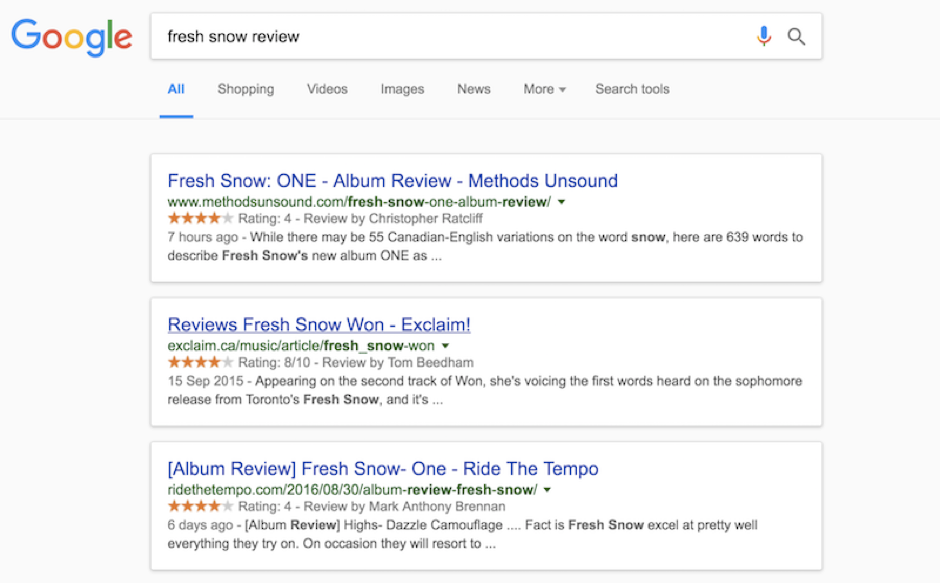A detailed, cleaned-up caption for the image could be:

---

This screenshot displays the Google homepage with a search for "Fresh Snow Review" entered in the search bar. The 'All' tab is selected underneath the search bar, with options for Shopping, Videos, Images, News, More, and Search Tools also visible.

Highlighted search results include:

1. **First Result**:
   - Title: "Fresh Snow 1 Album Review - Methods Unsound"
   - URL: "unsound.com/fresh-snow-1-album-review"
   - Rating: Four stars
   - Reviewed by: Christopher Ratcliffe
   - Published: Seven hours ago
   - Synopsis: Despite there being 55 Canadian English variations for the word 'snow,' Christopher Ratcliffe uses 639 words to describe Fresh Snow's latest album, "1."

2. **Second Result**:
   - Title: "Reviews: Fresh Snow 1" 
   - URL: "exclaim.ca/music/article/fresh_snow-1"
   - Rating: Four stars (8 out of 10)
   - Reviewed by: Tom Beatom
   - Published: September 15, 2015
   - Synopsis: The review notes that the sophomore release from Toronto-based band Fresh Snow starts with the voice of a female vocalist on the second track and continues to explore new sonic territories.

3. **Third Result**:
   - Title: "Album Review: Fresh Snow 1 - Ride the Tempo"
   - URL: "ridethetempo.com/2016/08/30/album-review-fresh-snow"
   - Rating: Four stars
   - Reviewed by: Mark Anthony Brennan
   - Published: Six days ago
   - Synopsis: Mark Anthony Brennan highlights that Fresh Snow excels in various musical endeavors, although occasionally they might employ familiar techniques (noted with ellipses).

---

This caption captures the essence of the search results related to reviews for Fresh Snow's album "1," providing an informative and visually descriptive narrative.